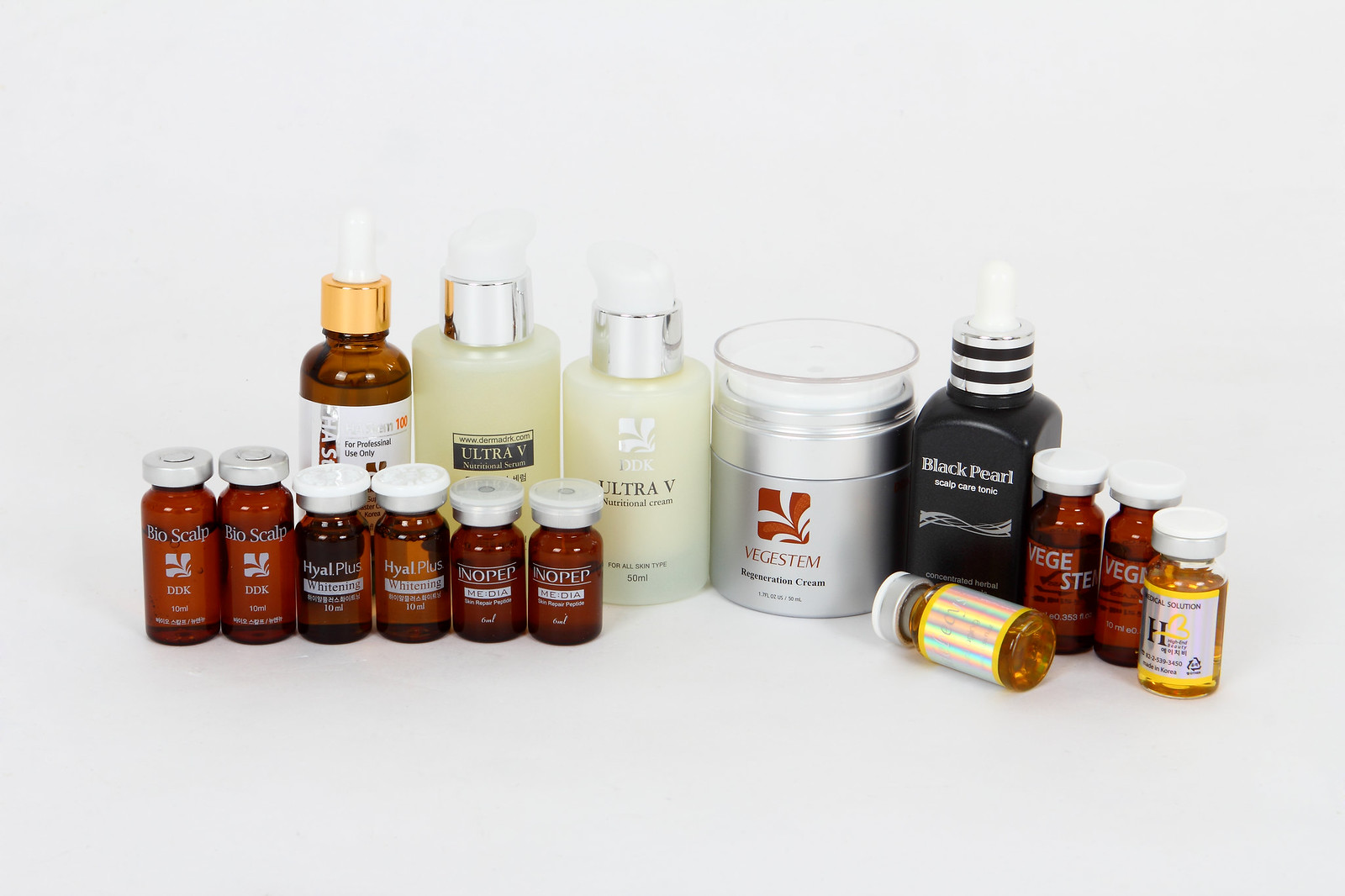The image features a white background that seamlessly blends with the primary visual component, rendering any lines or seams indistinguishable. At the forefront, there is an array of various products, some of which are identifiable as Dr. Scholl's, while others remain indistinct. The collection includes larger items and a diverse range of brands, with one product labeled "Here for Health" and another named "Black Pearl."

The majority of the bottles are brown with either brown or black labels. Among them, some have white labels designed to emulate a frosted glass appearance with a yellowish hue and are topped with silver caps. Notably, one silver bottle features a transparent cap, while the "Black Pearl" product stands out, with its black bottle adorned with white and black horizontal stripes around the lid.

In the midst of the collection, one bottle lies on its side, displaying either nutritional information or contents. This brown bottle with a white cap lies face down beside three similar bottles adjacent to the "Black Pearl." The products, possibly belonging to the beauty or nutritional supplements category, are arranged haphazardly yet collectively, creating a casual but organized display.